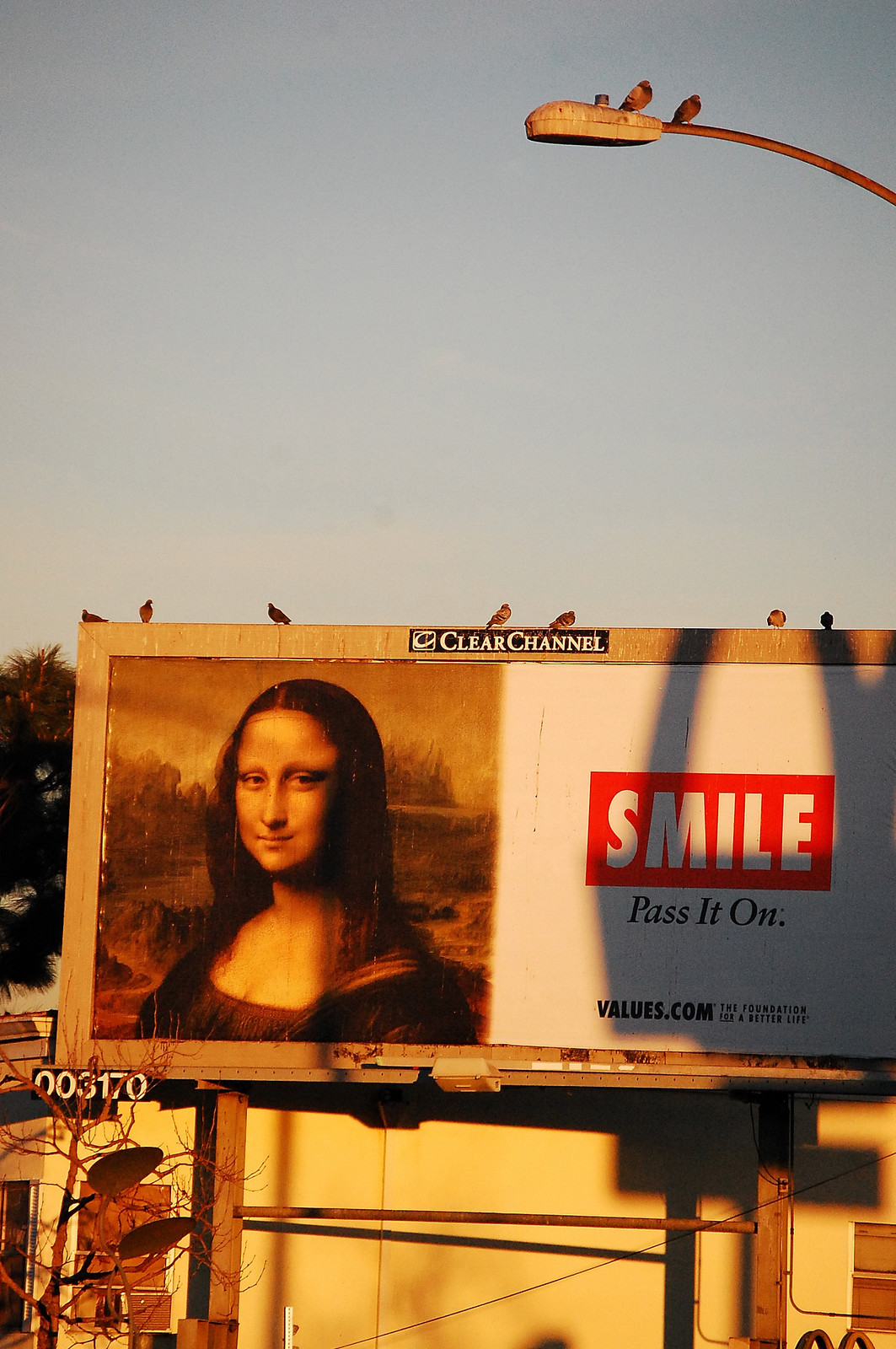This high-quality photograph captures a billboard mounted on a tan pole. Topping the billboard, text reads "Clear Channel" in black font against a white background. The billboard is split into two parts: the left side features a rendition of the Mona Lisa, while the right side displays a white background with a bold red and white sign that reads "Smile." Below the sign, text in black font says "Pass it on" followed by a website address, "blackvalues.com." Perched atop the billboard are several birds. This scene is set against a backdrop of a white building, on which some numbers are visible. In front of the building stands a small tree, and shadows cast on the wall further enhance the depth of the image.